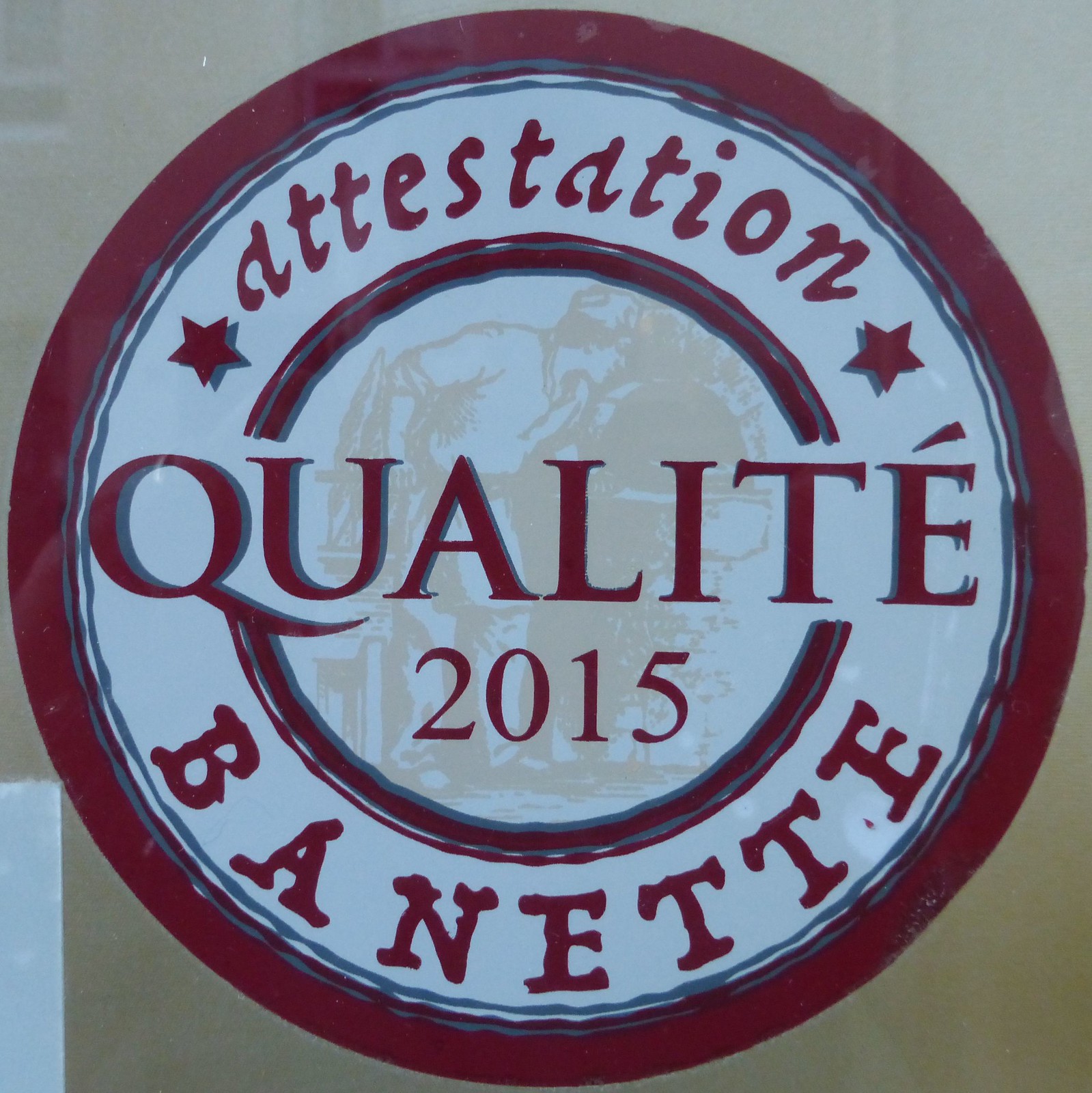In the image, we see a large circular logo centrally positioned against a light brown or tan background, with no other objects present. The outer border of the logo is a deep burgundy or maroon, followed by concentric borders in green, burgundy, white, gray, and then another white circle enclosing the main elements of the logo. At the center of the logo, there is a light tan illustration of a person, likely engaged in an undefined activity resembling work at a brick oven. The top semicircular section of the logo contains the text "Attestation," flanked by two burgundy stars. The middle section prominently features the words "Qualité 2015" in uppercase burgundy letters. At the bottom, within another semicircular border, the text "Banette" is displayed, also in uppercase burgundy letters. The font styles and sizes vary throughout the logo, contributing to its intricate design reminiscent of a certification or quality seal typically found on products.